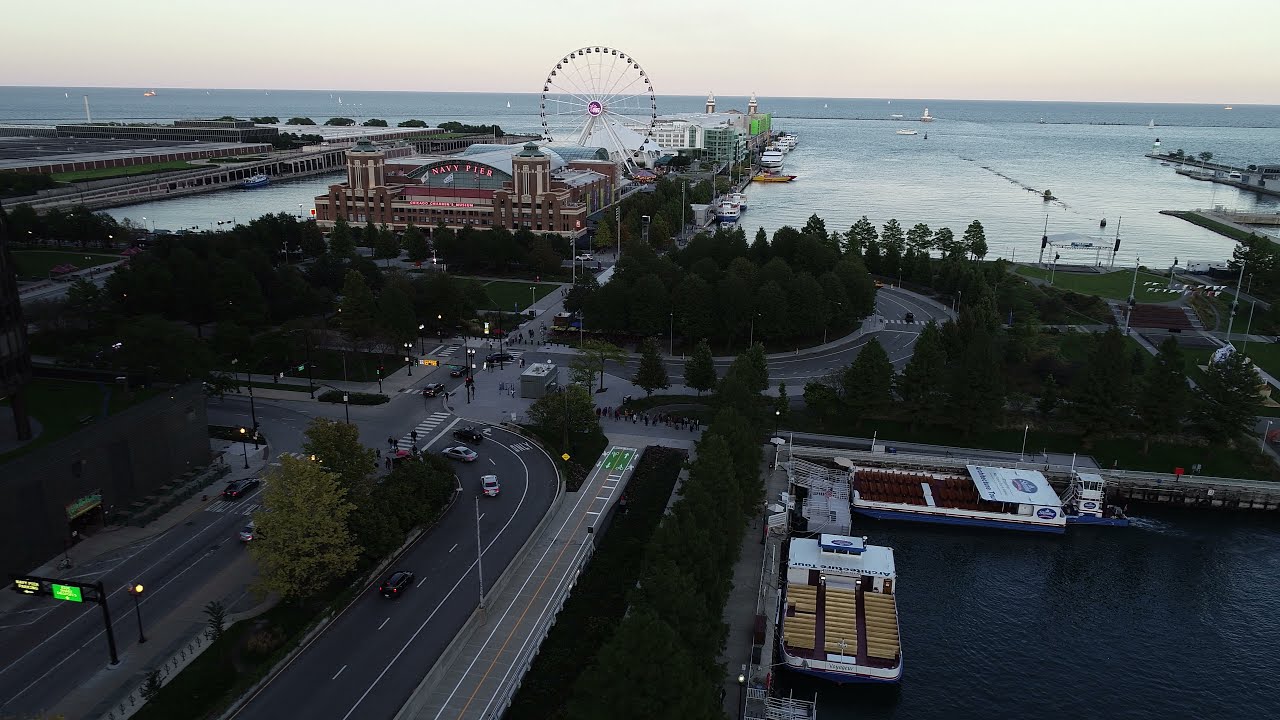The image captures an aerial view of a lively boat harbor featuring a distinct boardwalk dominated by a large Ferris wheel near a prominent older building labeled "Navy Pier." Surrounding the boardwalk is water on both sides, leading out to the open ocean dotted with numerous sailboats disappearing into a distant foggy horizon. Behind the boardwalk lies a cluster of hotel buildings extending toward the harbor, while the foreground showcases a bustling road network, including a sharp left turn leading to the boardwalk's entrance. To the right, the water harbors parked boats and larger hauling ships. The scene also includes a roundabout with cars navigating around it, set against a backdrop of a cloudy sky, suggesting the approach of evening.